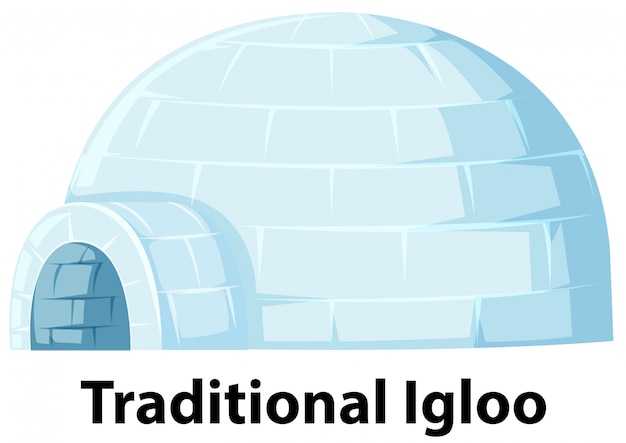The image is a stylized, computer-generated drawing of a traditional igloo, characterized by its classic dome shape made of large ice or snow blocks. The igloo features an arched entryway on the left-hand side, resembling the mouth of a pizza oven, through which one would crawl to enter the larger dome area. The igloo's surface displays a gradient of icy blue hues, transitioning from pale blue on the left to darker blue on the right, indicating a light source from the left. This color gradient is also evident in the entryway. Below the igloo, centered on a white background, is the text "traditional igloo" in bold black letters. The overall effect is a cliche yet detailed representation reminiscent of a cartoon image.